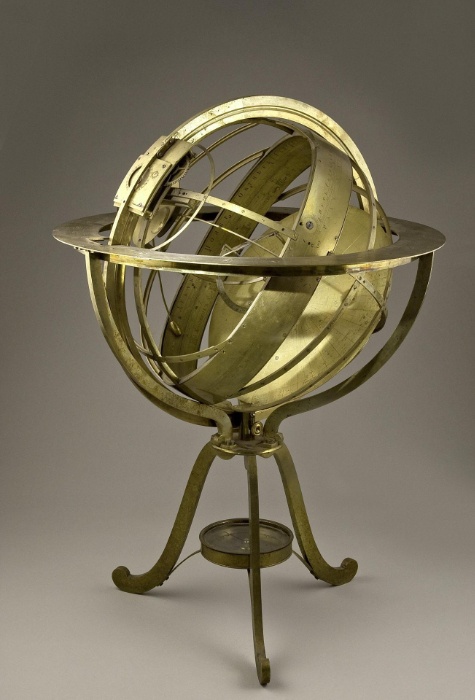This image shows a meticulously detailed piece of metalwork set against a grayish background that transitions into a slightly lighter hue at the bottom. The object's base comprises three brass-colored, curved metal legs. These legs support a thin metal pan designed to catch drips, suggesting it could hold a candle or catch oil.

Rising from the base, the legs converge to form a cage-like structure that encases a spherical, globe-like object. This sphere is composed of various metallic circular rings of different thicknesses and sizes, all designed to move independently on multiple axes, mimicking the motion of celestial orbits. The brass-like structure of the legs continues around the globe, which itself has openings, giving it an intricate yet sturdy appearance. The entire apparatus maintains a consistent dark yellowish, gold-toned color that is not overly shiny, lending an antique, well-crafted feel to the piece.